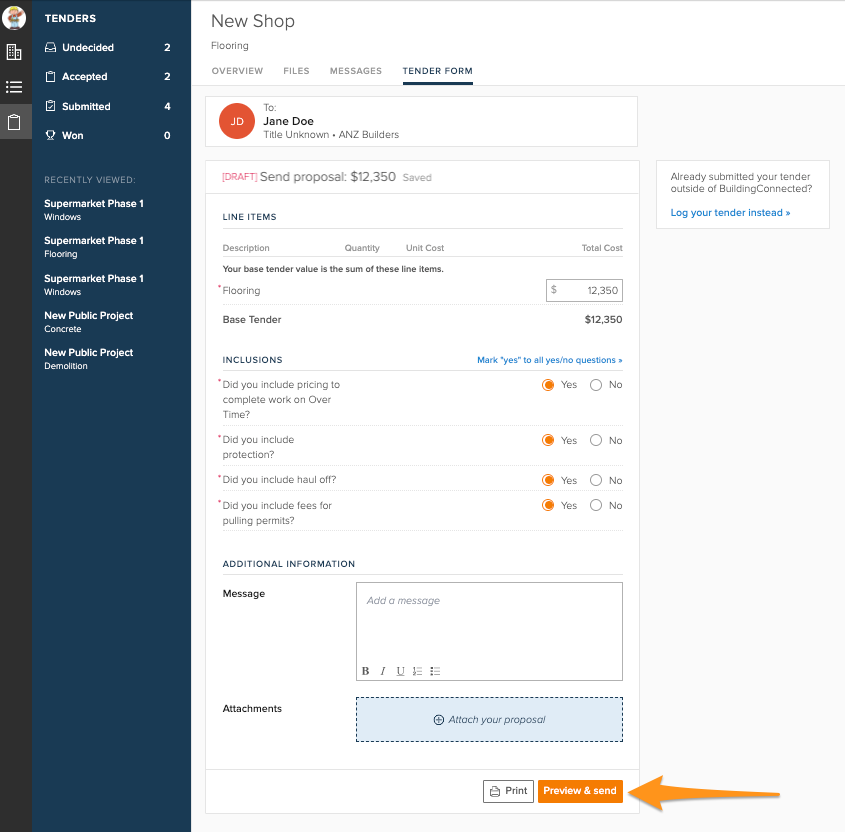A detailed screenshot of a website, presumably a website-building platform, showcasing a shop or business management interface. The primary color scheme features a dark navy blue background with white text for high contrast. On the left side of the interface, there is a navigation column that contains categories labeled "Undecided," "Accepted," "Submitted," and "Won," each with respective numerical indicators: two for "Undecided," two for "Accepted," four for "Submitted," and zero for "Won."

At the top left corner, there is a profile picture of a character resembling Bob the Builder with his left hand raised, set against a white background. Directly below the profile, there are several icons including a building logo, a hamburger menu icon, and a clipboard icon.

In the central area of the screenshot, the bolded text "New Shop" is prominently displayed, indicating the section where the user can initiate the creation or management of a shop. Above this section, the word "Forwarding" is written, possibly indicating a feature or tool in use. The user appears to be on a tab labeled "Tender Form," suggesting they are working on or viewing tender submissions or related documents.